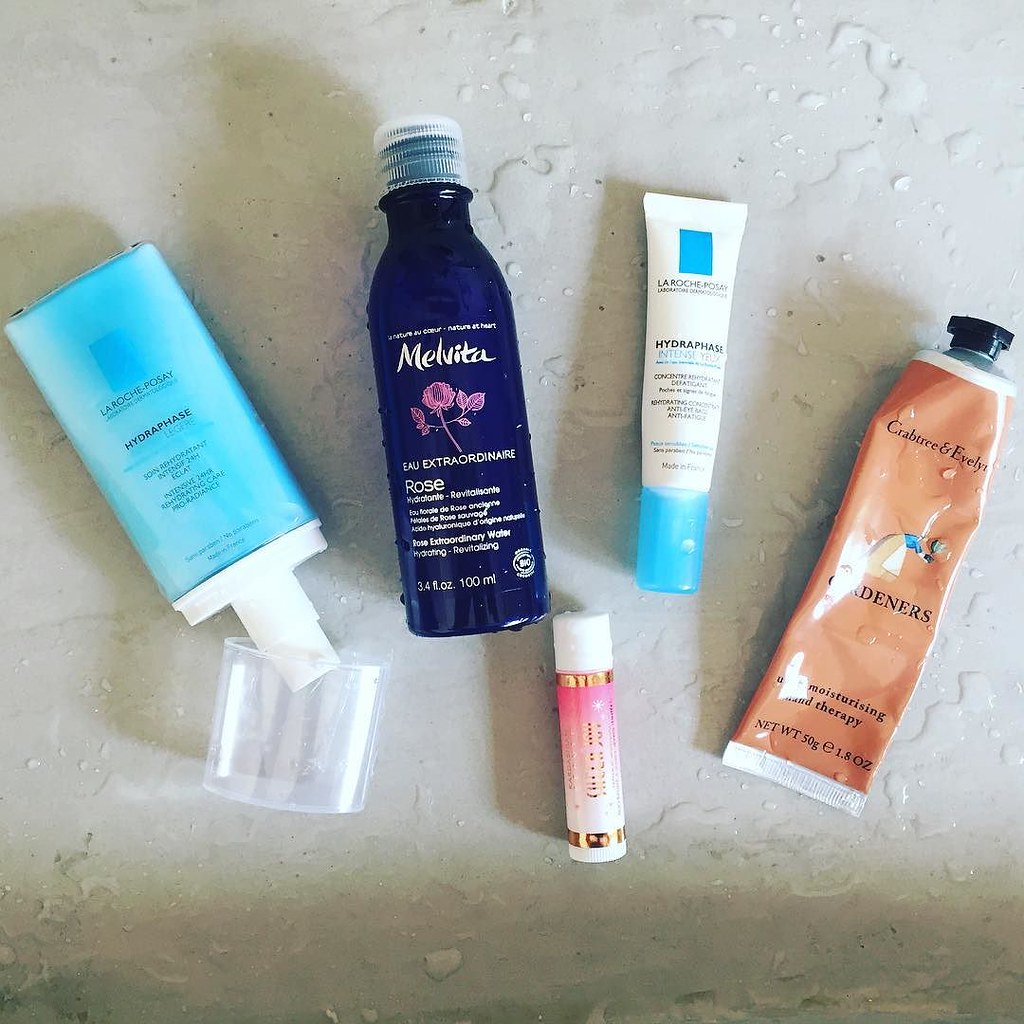This photograph captures a collection of skincare and cosmetic items arranged on a wet marble-tiled floor. The moisture on the floor is visible, adding a reflective sheen to the scene. On the center-left side of the image, there is a 1.8-ounce orange tube of Crabtree & Evelyn moisturizing lotion, which features an illustration of a woman. To its right, there is a smaller, 15ml tube of Hydraphase Intense by La Roche-Posay, characterized by its white body and light blue cap. Further to the right is a 3.4-ounce blue bottle of Melvita Eau Extraordinaire Rose lotion, adorned with a clear white cap. Adjacent to this, slightly to the left, is another La Roche-Posay product: a small spray bottle of Hydraphase, distinguished by its clear cap that has been removed. Below the Melvita bottle lies a pink-toned lipstick with a white cap. The composition of these items on the damp marble creates a delicate interplay of colors and reflections, adding to the atmospheric feel of the scene.